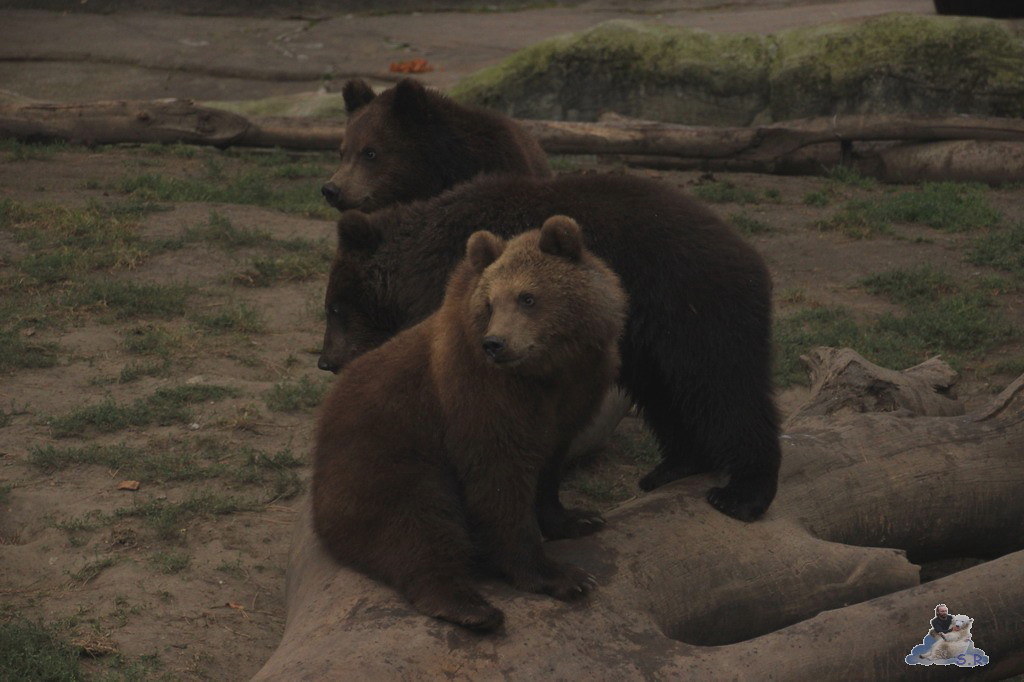In the image, there are three bears in a captivity setting with a primarily hard dirt ground, sporadically dotted with small green patches. Central to the scene is a large, fallen tree trunk running horizontally across the foreground. Sitting towards the right end of this trunk is a brown bear, its body oriented to the right while its head turns to the left, looking over its shoulder. Near this bear is a darker brown bear standing on all fours, also facing left. A third bear, slightly more brown than the second, stands further behind, also facing to the left. Surrounding this area, there are some green trees providing a natural yet confined backdrop, with a faint red truck visible in the distance.